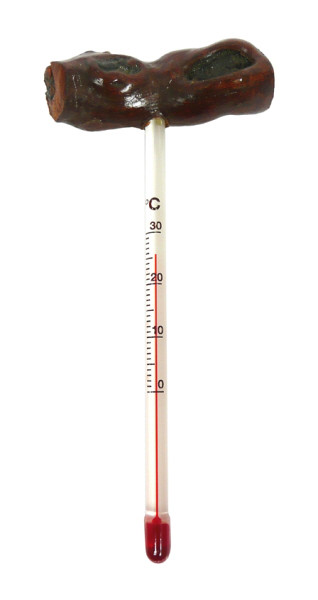The photograph captures a vintage glass mercury thermometer reminiscent of those used in 1950s doctor's offices. Positioned against a stark white background, the thermometer prominently displays Celsius measurements, with a distinct red mercury line indicating a temperature of approximately 25 degrees Celsius. Intriguingly, the top end of the thermometer is inserted into an unidentified object that is brown and black in color. This object, around two inches in length, has a shiny surface and an irregular shape. It evokes comparisons to various items, ranging from dark candy, like a Tootsie Roll or taffy, to organic materials such as wood or petrified bark, making its precise nature ambiguous but adding an element of curiosity to the image.